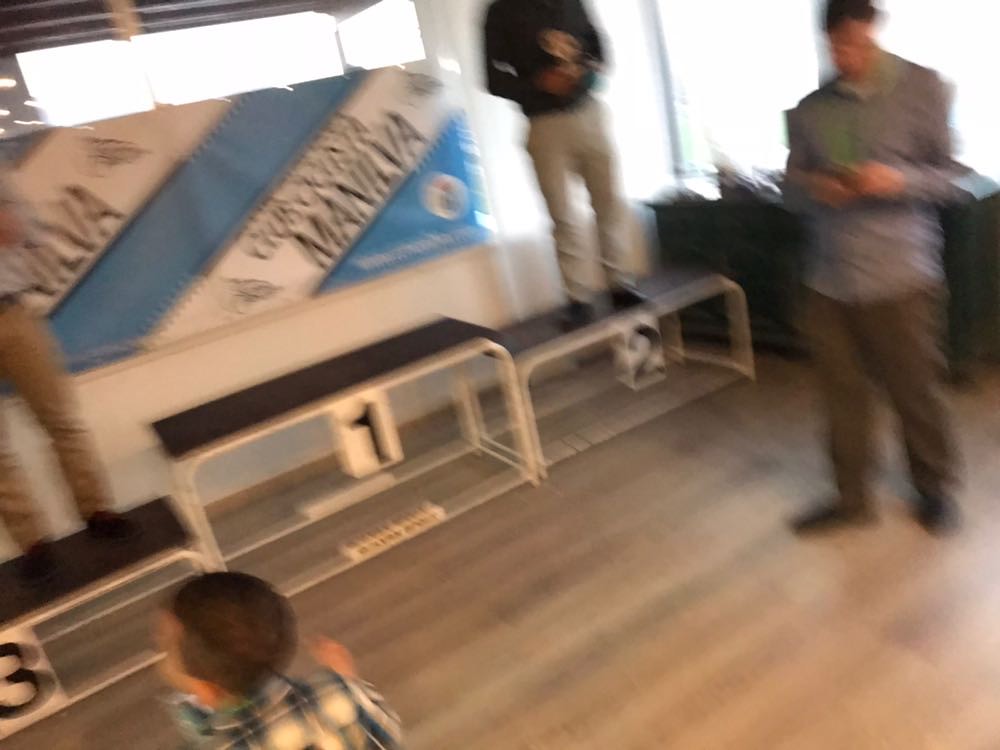This extremely blurry photograph captures an indoor scene featuring a competition award podium setup on a brown-to-gray hardwood floor. The podium, comprised of three black, tubular metal platforms of varying heights, is labeled with white rectangular plaques bearing the numbers 1, 2, and 3. The tallest podium, marked with a '1,' is centrally positioned, flanked by the shorter '3' on the left and the medium '2' on the right. Three figures stand on the podium: a man on the '2' platform, another man on the '3' platform, and the '1' platform possibly vacant. Additionally, in the lower left corner, a child in a blue and white plaid shirt is visible from the shoulders up. To the right, a man in brown pants and a brown or tan button-front shirt appears engrossed in his cell phone. The upper left corner reveals a white wall with a banner featuring baby blue and white 45-degree stripes and illegible black text, partially obscuring either a window or mirror reflecting or showing a blown-out white sky. The setting is characterized by a sense of motion, contributing to the blurred details and overall lack of sharp focus.